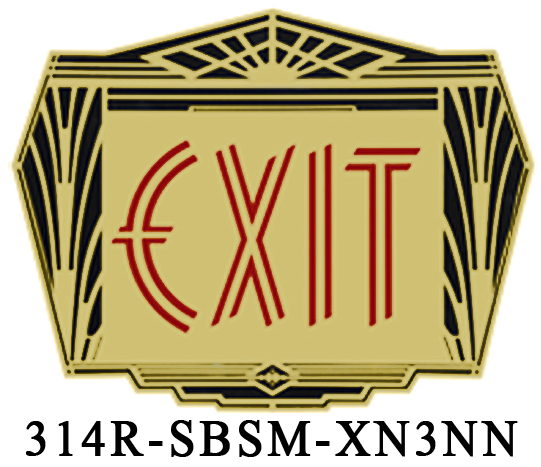This illustration depicts a vintage-style exit sign crafted in an ornate Art Deco design, possibly reminiscent of the 1920s or 1930s. The sign appears to be made of a gold-colored metal, accented with black trim around its edges. Central to the design, the word "EXIT" is prominently displayed in red, outlined letters. The upper portion of the sign features a rising sun motif that culminates in a diamond-shaped medallion at its base. Flanking the top are patterns resembling palm tree branches, adding to the intricate Art Deco aesthetic. The background is a beige or cream hue, providing a contrasting backdrop for the bold design elements. Below the diamond-shaped medallion, a product number "314R-SBSM-XN3NN" is distinctly inscribed. This decorative exit medallion would be fitting for a fine or luxurious Art Deco hotel, enhancing the elegance of an exit doorway.